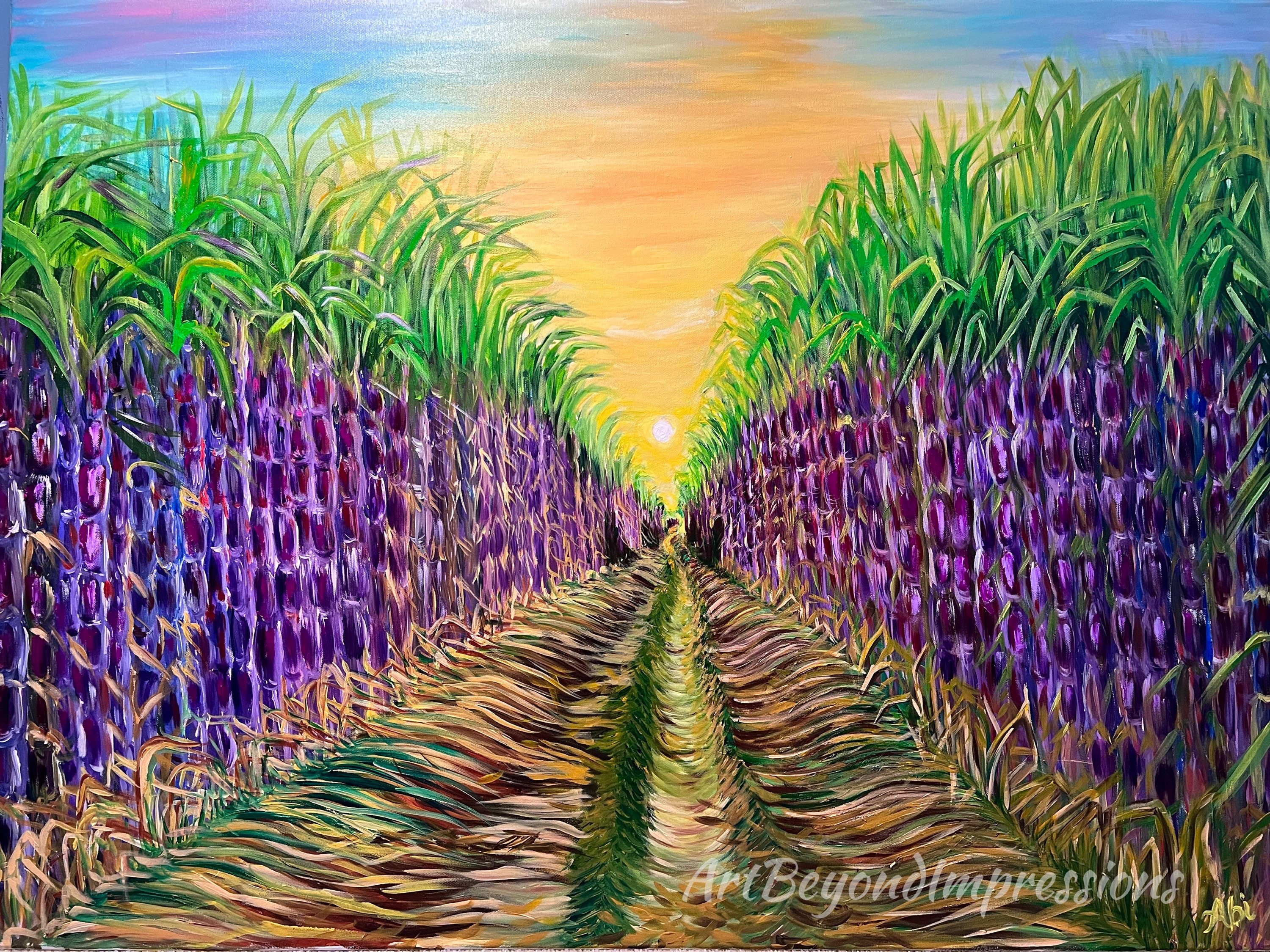This vivid painting depicts a vibrant scene of a cornfield at sunset, divided into a harmonious nine-point grid. The composition is anchored by a central pathway that appears to be a recently harvested row, narrowing as it extends into the distance. On either side, tall, unharvested corn stalks stand prominently, their stems rendered in striking purples and blues, topped with lush green leaves. The golden husks contrast beautifully against the foliage. The sky above is a breathtaking gradient of colors, transitioning from bright yellow near the peeking sun to soft hues of orange, pink, and blue, capturing the essence of a serene sunset. In the bottom right corner, the painting is marked with a light stylized font that reads "Art Beyond Impressions," along with a slightly yellow signature bearing the initials "A.B.I." This detailed composition not only highlights the intricate textures and colors of the cornfield but also evokes a sense of tranquility and natural beauty.